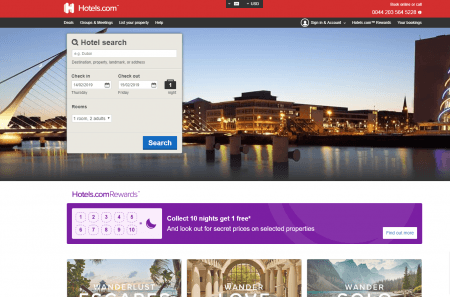The top portion of the image features a clean white background. On the left side, "Hotels.com Rewards" is prominently displayed in purple font, with both "Hotels" and "Rewards" beginning with capital letters. Below this, a purple rectangle spans the width of the image, containing a smaller white rectangle on its left side. Inside this white rectangle are ten small, dotted squares organized into two rows and filled in purple from numbers one to five on the top row and from six to ten on the bottom row.

Adjacent to this, the text "Collect 10 nights and get 1 free" appears next to a purple crescent shape. Further down, there is some text mentioning "secret prices" available on specific properties, but it is largely unreadable due to blurriness. A white rectangle below this possibly says "Find out more," but the text lacks clarity.

At the bottom of the image, there are three distinct pictures. The leftmost image displays a beach scene and is captioned "Wanderlust." The middle image showcases what appears to be a Greek column with the caption "Wanderlust." The image on the right portrays a woodland setting and features the caption "Wander slowly."